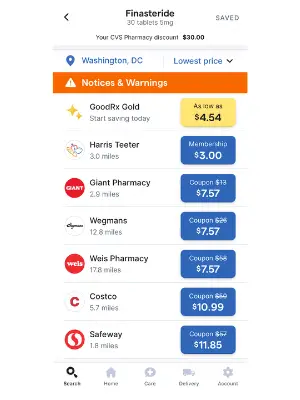The image depicts a comparison chart on Finasteride pricing, featuring CVS Pharmacy discounts in Washington, D.C. The chart is slightly blurred with a white background and an orange bar at the top. A white triangle with an exclamation mark in it is present at the top-left corner, indicating warnings or notices. The chart lists prices from various pharmacies: GoodRx Gold at $4.54, Harness & Teeter at $3, Giant Pharmacy at $7.57, Wegmans at $7.57, Weiners Pharmacy at $7.57, Costco at $10.99, and Safeway at $11.85. Additional elements include non-price-related text such as "Roerwijk," "Search," "Home," "Store," "Getaway," "Janelle," and "the bottom." These words are rendered in gray at the bottom of the image.